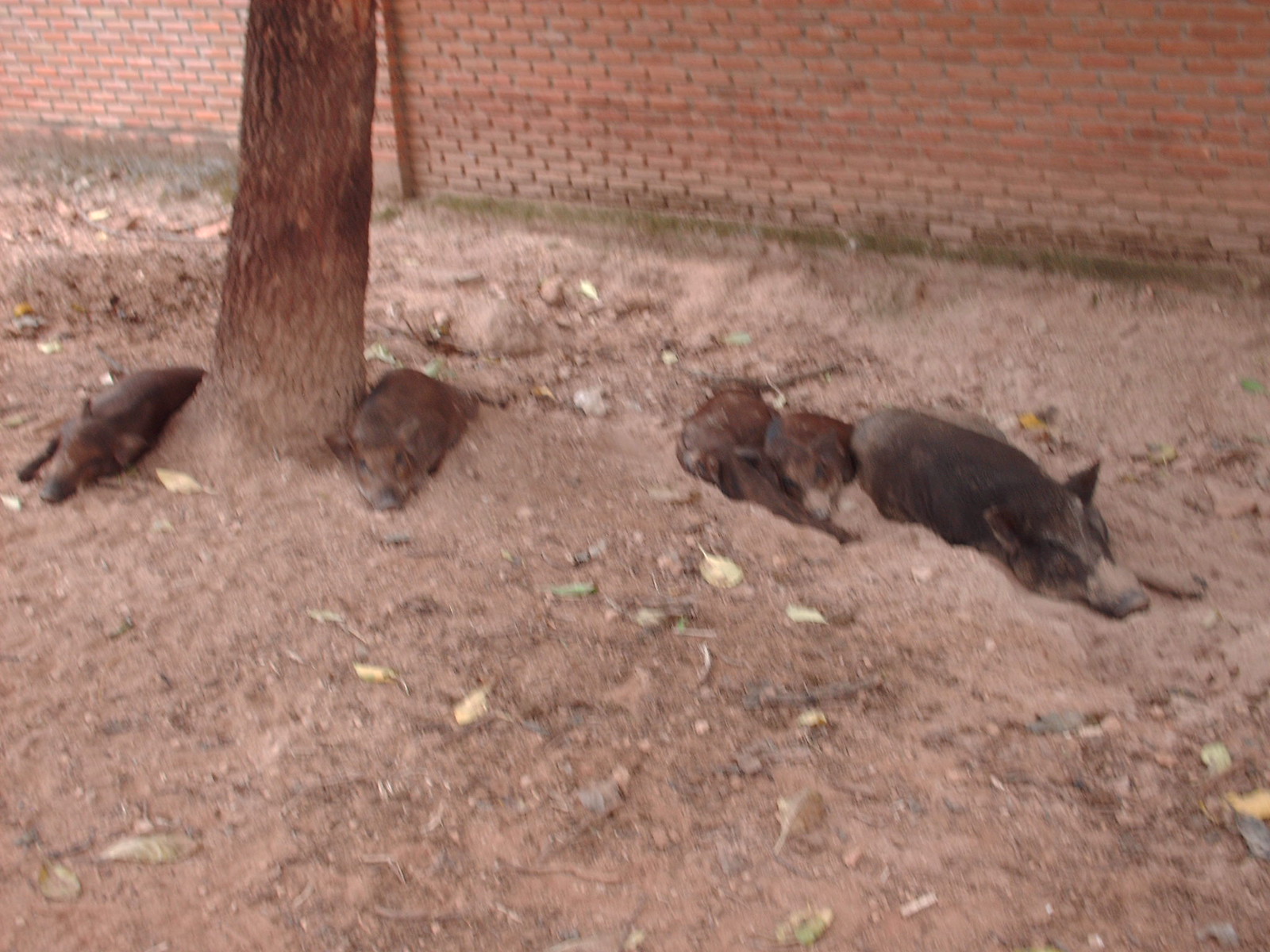This is a color photograph taken outdoors with an orangey-red filter applied, giving it an overall warm hue. In the foreground, there's ground covered with orangey-red dirt, interspersed with pale yellow and green leaves and some twigs, possibly from the tree above. To the left stands a tree trunk, around which a group of five wild pigs, or boars, are reclining. These pigs are dark brown in color and vary in size, suggesting a mix of adults and possibly younger pigs. One pig's head and snout are visible to the right of the tree, although it's challenging to identify the species clearly. The pigs appear to be resting in the dirt to keep cool. Behind the tree trunk runs a thin green line of moss, which intersects a red brick wall extending from the top right to the top left of the image. The bricks are mostly uniform in color, though the bottom ones appear discolored, with shades of dark greenish-brown and pale patches.